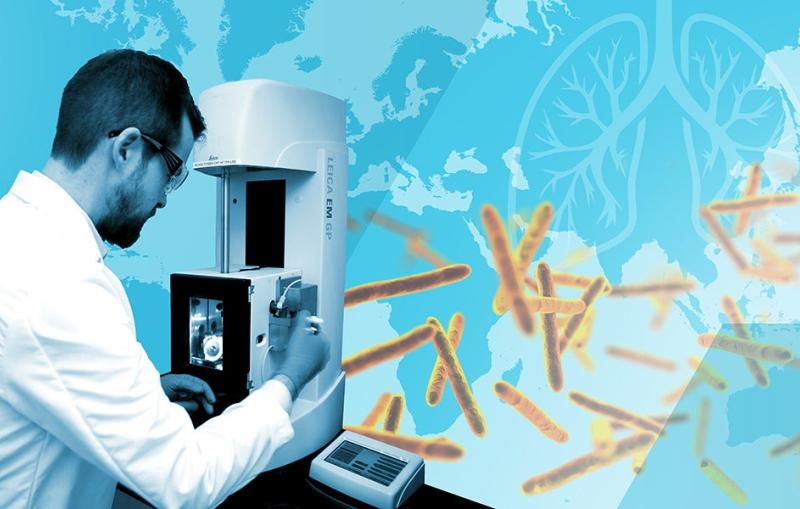In the image, we see a scientist deeply engrossed in his work within a well-equipped laboratory. He is examining a specimen using a sophisticated device, likely an electron microscope, identifiable by the name “Leica EMGP” on its side. The scientist, characterized by his brown hair, beard, and mustache, and wearing a white lab coat and safety glasses, stands at a black tabletop with his hand interacting with various components of the microscope. Notably, this complex apparatus features a central panel with gears to adjust the specimen's position and a large chamber with a visible window, illuminated from within, allowing intricate observation.

To the right, a smaller machine sits, while to the left, the large chamber showcases a metal pole extending through its top into a white-capped component above. The image is artistically enhanced with a creative background that includes an illustration of human lungs, stylized depictions of bacteria in red, yellow, and orange, and a blue and white representation of the globe. These elements hint at the scientific and possibly medical nature of the research, merging real and illustrative visuals to convey the broader impact of the scientist’s work.